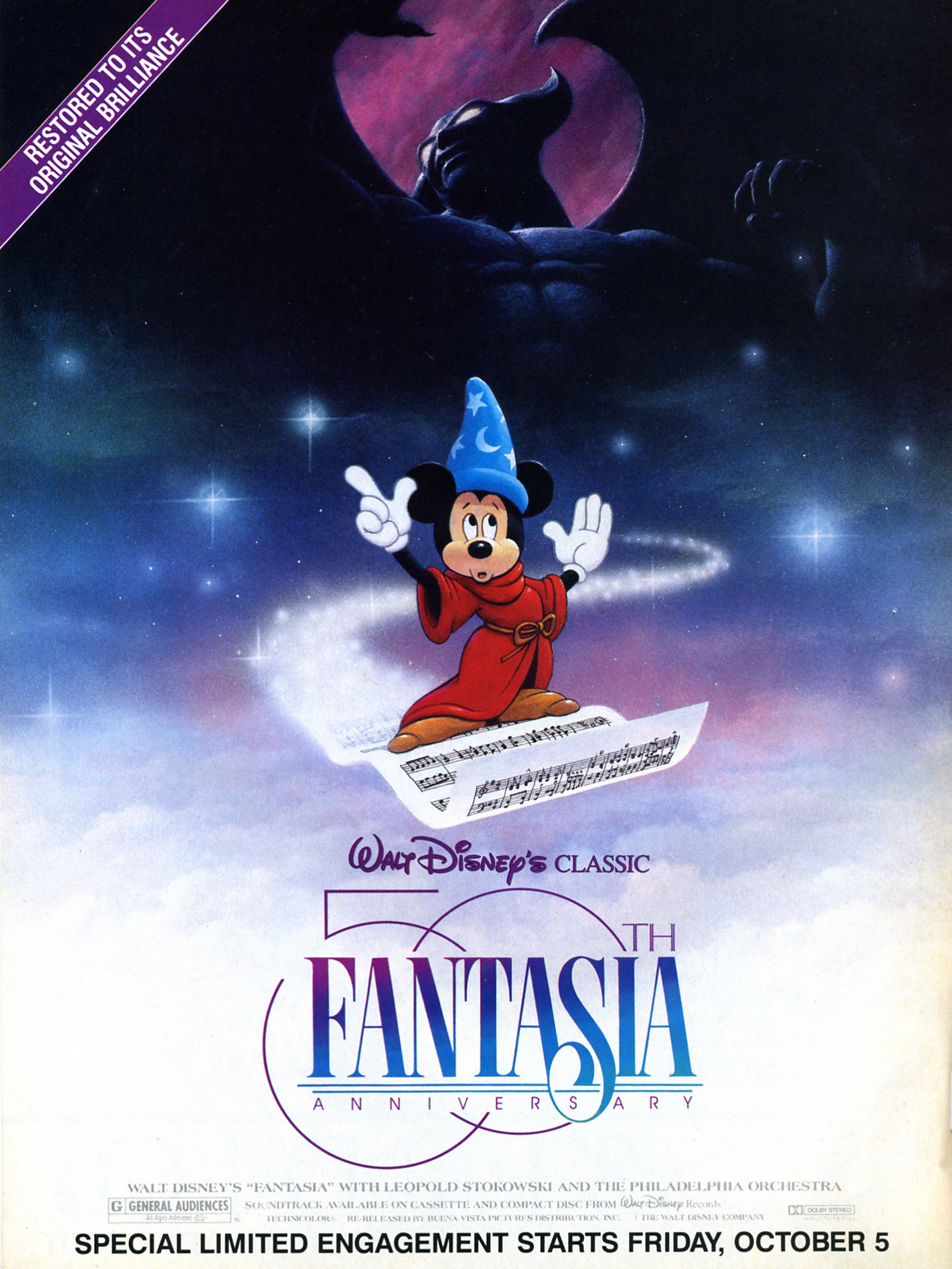The image is a vibrant advertisement for a publication celebrating the 50th anniversary of Walt Disney's classic film, "Fantasia." At the forefront, the beloved cartoon character Minnie Mouse is depicted with her iconic black ears, sizable white gloves, and black arms. She's adorned in a red robe, cinched at the waist, and is wearing large brown shoes. Minnie stands poised as if she is riding a sheet of music like a magic carpet, soaring above the clouds. The background is a deep blue sky filled with scattered stars, adding to the enchanting atmosphere.

In the backdrop, a menacing, dark character with wings and glowing yellow eyes looms ominously, spanning the entire width of the image. This character heightens the dramatic effect of the scene, contrasting with Minnie's vibrant appearance.

In the top right-hand corner of the image, the text reads, "Restored to its original brilliance." Below Minnie Mouse, there is additional text that states, "Walt Disney's classic 50th Fantasia anniversary." At the bottom of the image, there's further information about the film, including the release announcement in bold black letters: "Special limited engagement starts Friday, October 5."